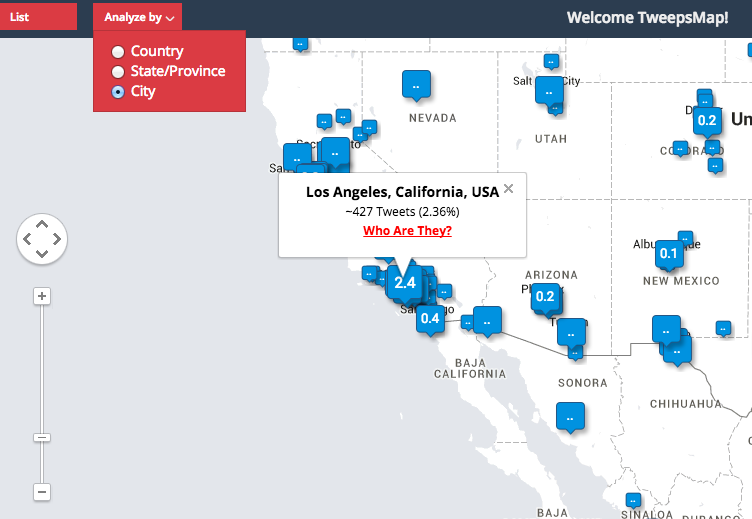Screenshot of a Navigational Map Interface

The presented image is a screenshot from a computer displaying a detailed navigational map interface. At the top of the screenshot, there is a navy-colored navigation bar. This bar includes a red button labeled "List" and another button titled "Analyzed by," accompanied by a drop-down menu with three options: Country, State/Province, and City. The city option is currently selected, indicated by a filled circle.

To the right of these buttons, the bar displays the text "Welcome to Tweepsmap." The map itself shows the southwestern region of the United States and parts of Mexico, including California, Nevada, Utah, Colorado, New Mexico, and Arizona. The map also highlights regions in Mexico such as Baja California, Sonora, and Chihuahua, with partial visibility of Baja California and Sinaloa at the bottom.

Blue speech bubble icons, some containing numerical values, are scattered throughout the map, signifying different data points. Hovering above Los Angeles, California, is a pop-up information box. This rectangular box shows detailed statistics including, "Los Angeles, California, 427 tweets (2.36%)." The phrase "Who are they?" is displayed in underlined red text, implying a clickable link. The pop-up box also features a small "X" icon for closing the window. The bubble indicator on the map corresponding to this pop-up displays "2.4."

This screenshot offers a detailed and interactive representation of tweet distribution across the specified regions.